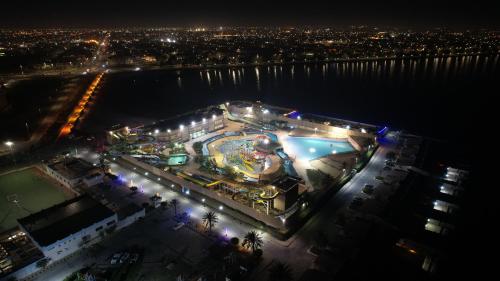This photograph captures a brightly-lit, square-shaped waterpark and resort area at night, viewed from an aerial perspective at an altitude of approximately 100 to 200 feet. The centerpiece is a well-illuminated pool surrounded by multiple water slides, hot tubs, and various other water attractions, conveying a vibrant nighttime atmosphere. Adjacent to the pool is a two-story building, possibly a hotel or clubhouse, integrated within the park's confines. Surrounding the square are palm trees, parking areas with discernible cars, and a sports field, possibly for tennis or basketball. To the left side of the image, there's a road and a bridge that connects the resort area to a sprawling cityscape visible on the horizon. The lights from the distant city contrast against the dark night sky, while a large, dark body of water lies between the waterpark and the row of distant buildings, further enhancing the photograph's depth and detail.